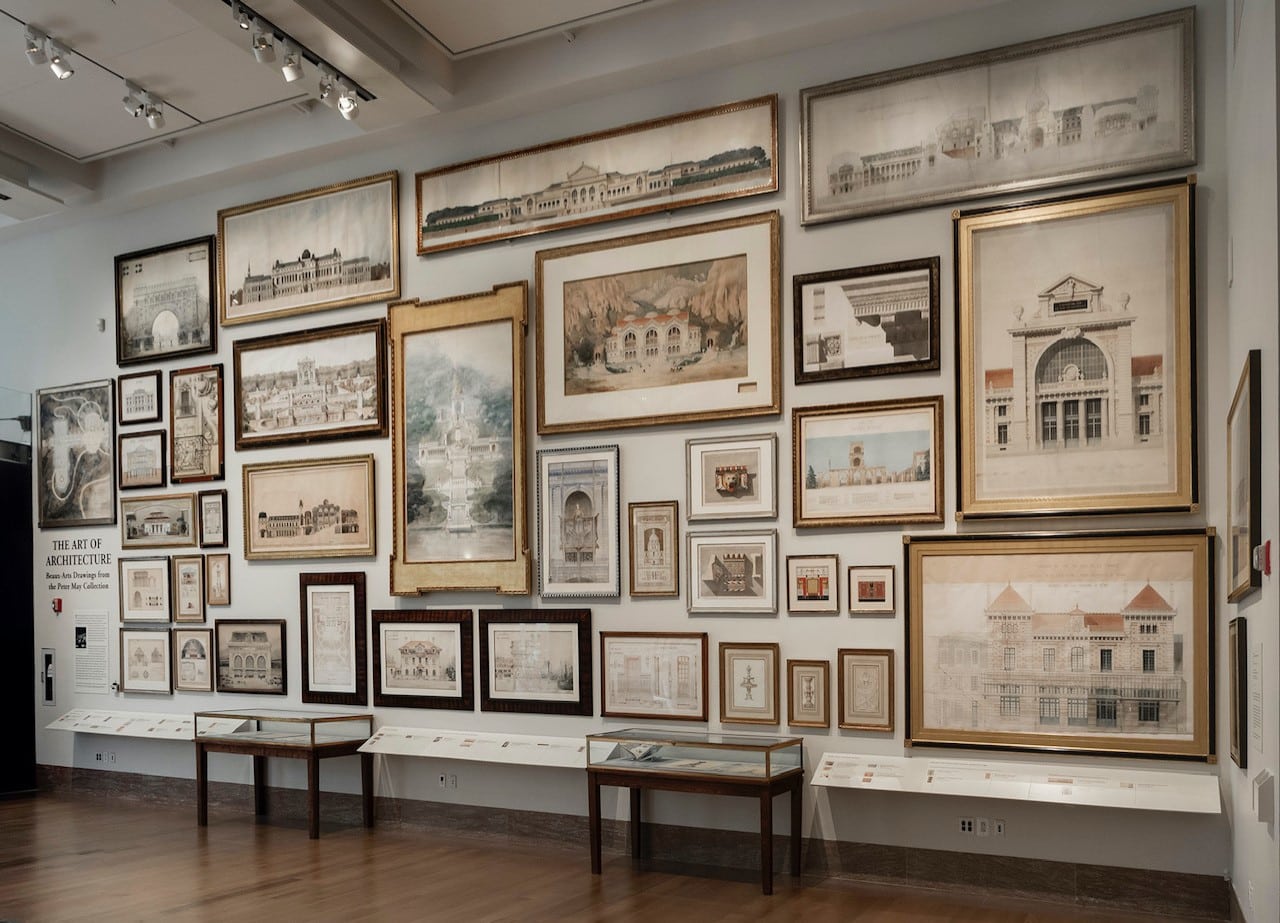The image depicts a museum or art gallery room with a light-colored, pale gray wall adorned with various framed pictures and drawings, predominantly of buildings. The frames are diverse, including golden, black, and wooden ones, and vary in size from very large to small, even coffee-table-sized artworks. The wall spans approximately 10 feet in height and 20 feet in length, featuring a systematic arrangement: larger frames on the top, middle, and right side, and smaller ones on the left and bottom sections. 

The upper left corner showcases multiple light fixtures affixed to the ceiling, illuminating different parts of the gallery. A slight section of the ceiling is visible, particularly where the lighting is directed. On the left side of the image, around the middle or slightly lower, there is a doorway that extends off the image. Adjacent to the main wall on the right side is another wall with a couple of wall hangings positioned lower on it.

In front of the main wall are several brown, wooden display tables with glass tops, each supported by four legs. These tables are positioned between ledges that protrude from the bottom of the wall, potentially holding informational writing. The floor of the room is a rich, dark brown hardwood, adding warmth to the exhibit space.